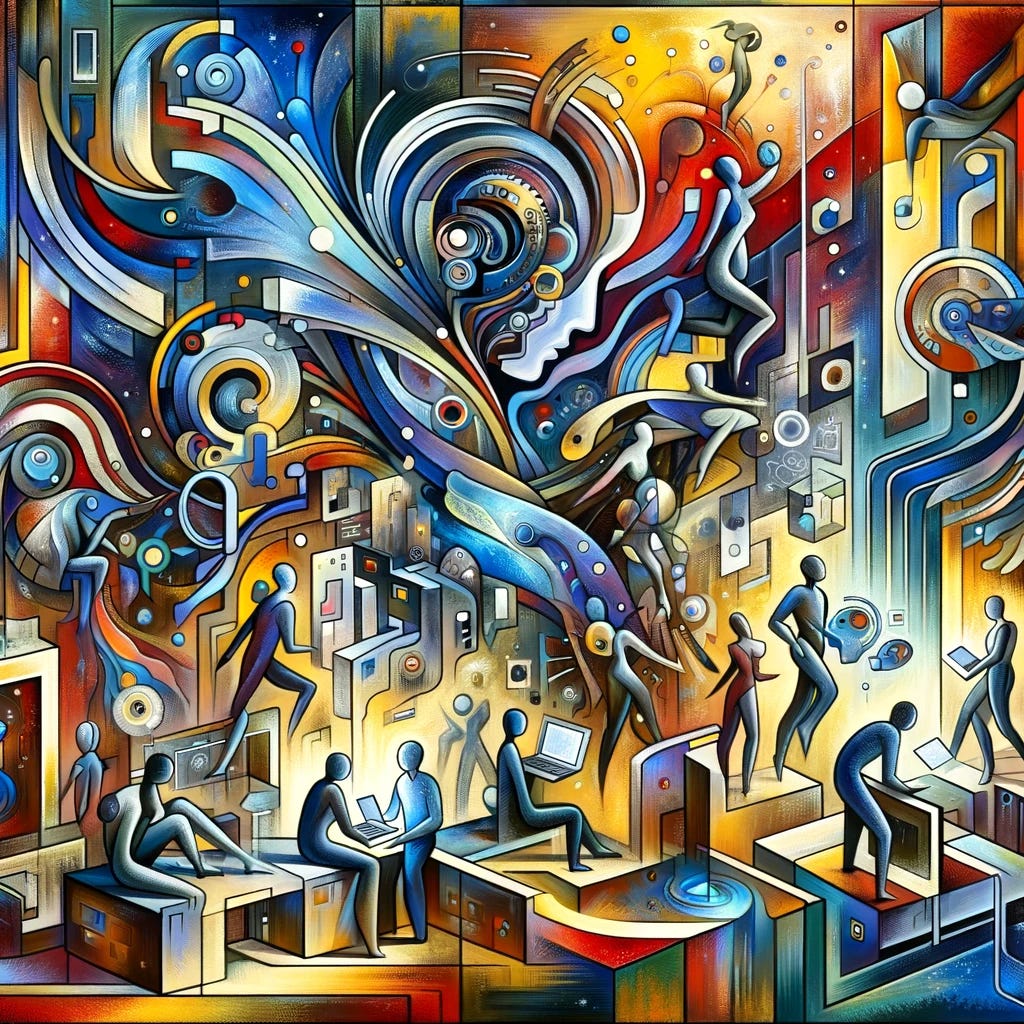This image is a square, six-inch high by six-inch wide piece of art, done in an artistic impressionist style. It is a chaotic yet vividly detailed drawing with rich colors such as blues, reds, purples, and golds. The background features a wall that occupies the majority of the upper part of the image, filled with patterns in aforementioned colors, creating a visually stimulating backdrop.

At the center top, a side profile of a human head is depicted, opened up to reveal intricate gears and mechanical components inside, symbolizing a blend of human thought and machinery. Surrounding this focal point are numerous faceless, humanoid figures with indistinctive features, rendered in shades of blue, brown, purple, and red. These figures are scattered throughout the composition, holding or interacting with various futuristic technological devices like laptops, tablets, cell phones, and headsets.

Towards the bottom of the image, more recognizable and detailed elements emerge. There is a depiction of a work desk with a person seated at it, another couple engrossed in a book, and a third person focused on a laptop. Additional figures are seen dancing or walking, adding to the dynamism of the scene. Some figures are even hovering in the air, holding spherical objects or small dots in their abstracted hands.

The overall impression is one of a frenetic, technology-infused environment, where human forms and mechanical elements coexist in a vibrant, surrealistic tableau.